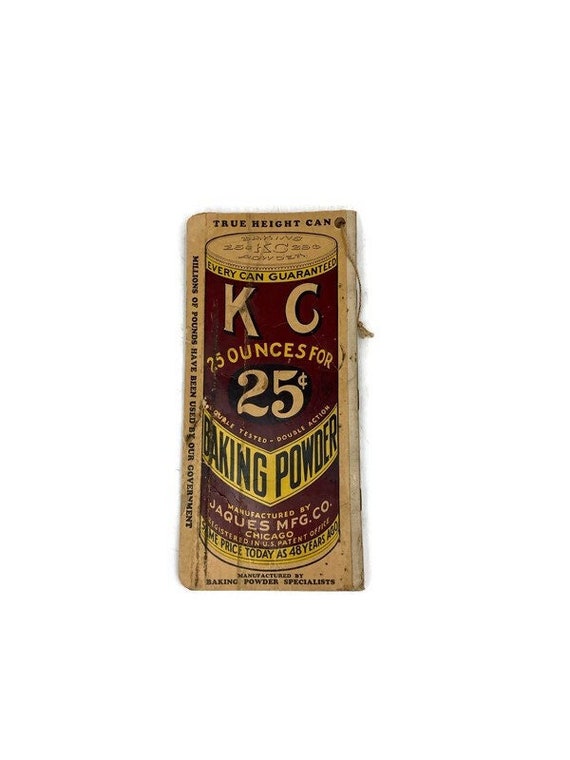The image displays an antique advertisement for KC Baking Powder, prominently featuring a red and yellow depiction of the can, which claims the same price of 25 cents for 25 ounces as it had 48 years prior. The text highlights the qualities of "tested double action" and assures "every can guaranteed." The advertisement, manufactured by Jacques MFG Co. in Chicago, is presented on a flat piece of wood with hanging capability, with intricate details etched and colored in black and white. This vintage piece not only promotes the product but also serves as a charming historical artifact, suitable for display on a keychain or hook.